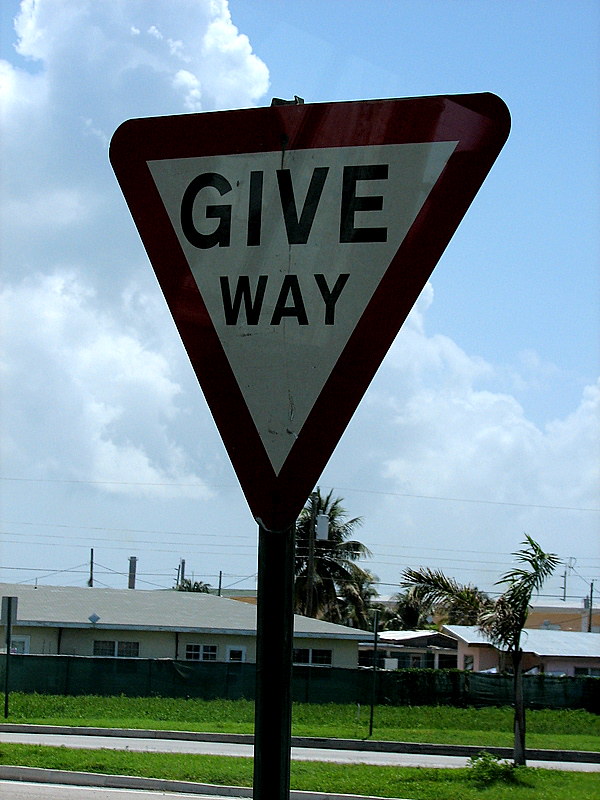In this outdoor photograph, the primary focus is a large street sign mounted on a black post. The sign, an upside-down triangle typical of a yield sign, instead displays the words "Give Away" in black lettering on a white background. Beyond the sign, a residential neighborhood comes into view, characterized by well-maintained green grass and fencing, suggesting the photograph is taken from the backside where the neighborhood meets the street. The street below the grassy area further indicates this boundary. Rooftops of various houses peek into view, affirming the residential setting. The presence of palm trees hints at a warm climate, all under a bright blue sky scattered with a few clouds, adding to the overall picturesque quality of the scene.